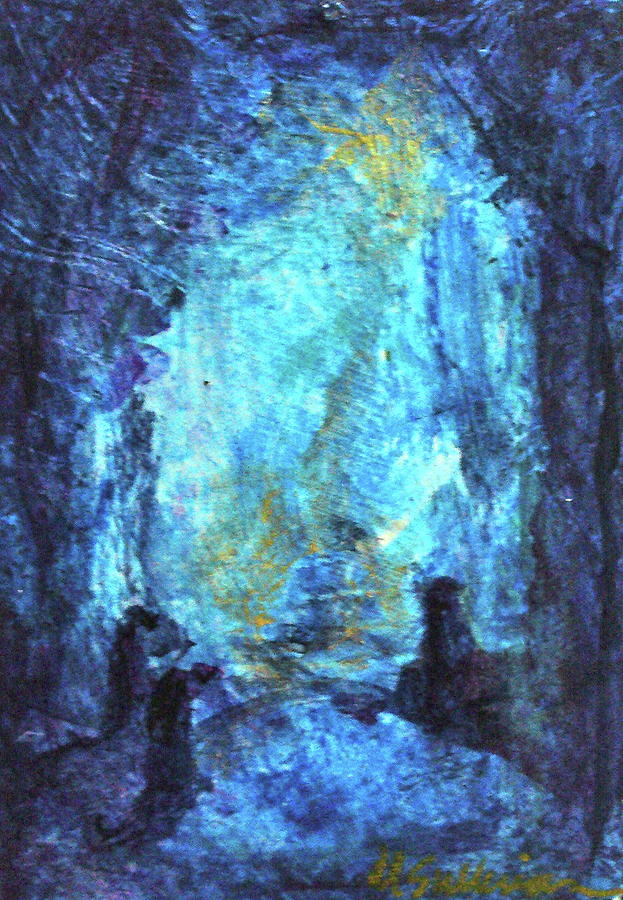This detailed and abstract contemporary painting, standing upright and rectangular in shape, is predominantly composed of varying shades of blue—from deep, shadowy dark blues around the edges to lighter, almost ethereal blues in the center. Subtle hints of purple, yellow, and white add depth and contrast to the composition. 

In the upper middle part of the painting, a yellow highlight suggests the presence of a sun, casting a subtle trail of light that seems to descend towards the bottom of the image. This light creates an impression of an opening or a clearing within the scene, evocative of an entrance to a cave or a mystical realm.

At the bottom of the painting, three dark-colored figures with elongated snouts and visible tails, resembling panthers or similar animals, are positioned in a triangular formation. These figures appear to be sitting or standing on all fours, intently gazing towards the central light source or structure, creating a sense of anticipation or worship.

The overall effect is both mysterious and mesmerizing, as the swirling colors and indistinct shapes blur the lines between reality and abstraction. This captivating painting, enigmatic in its intent, is signed by its artist in the lower right corner, adding a personal touch to the hauntingly beautiful composition.